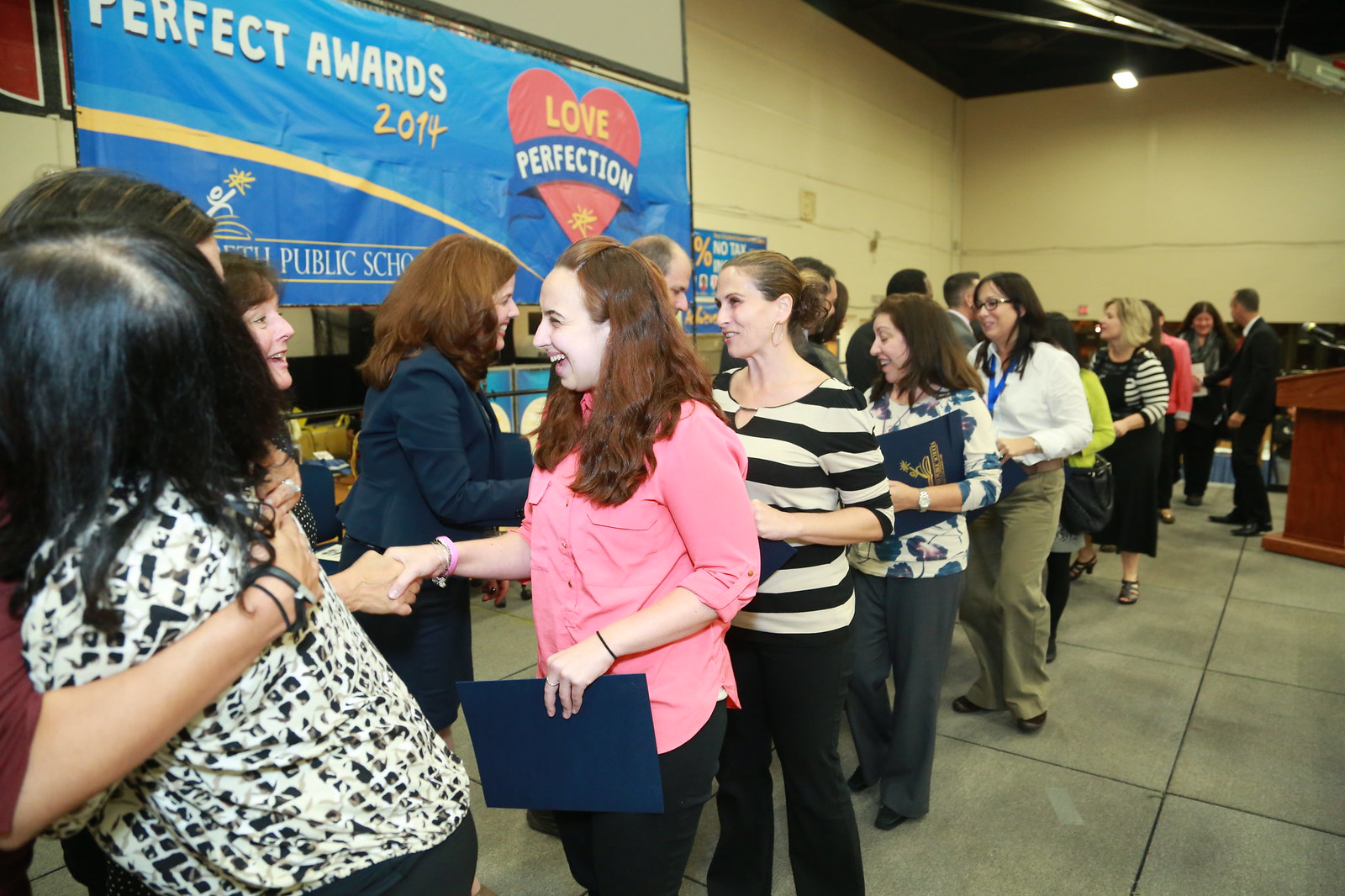Inside a spacious warehouse or gym, a significant gathering unfolds, showcasing a long line of predominantly female attendees, estimated at around a dozen or more, all dressed in business casual attire, with some in dresses. These individuals are part of the "Perfect Awards 2014" event, as revealed by the blue banner draped on the back wall, emblazoned with a red heart featuring "Love" in yellow and "Perfection" on a sash around the heart, along with text for "public schools" partially obscured. The atmosphere is warm and engaging, with many participants smiling and actively shaking hands as they progress down the line towards a presentation area marked by a podium on the right. In the foreground, on the bottom right, a poignant moment of a woman with long dark hair and a black-and-white patterned shirt being hugged by another woman in a brown top adds a personal touch. Behind them, another pair of women, one in pink, are shaking hands, further emphasizing the collaborative spirit of the event. Lining up to meet the greeters, many participants hold blue binders featuring gold insignia, possibly related to the awards being presented. The scene captures a celebration of recognition, likely honoring teachers for their dedication and service in public schools.